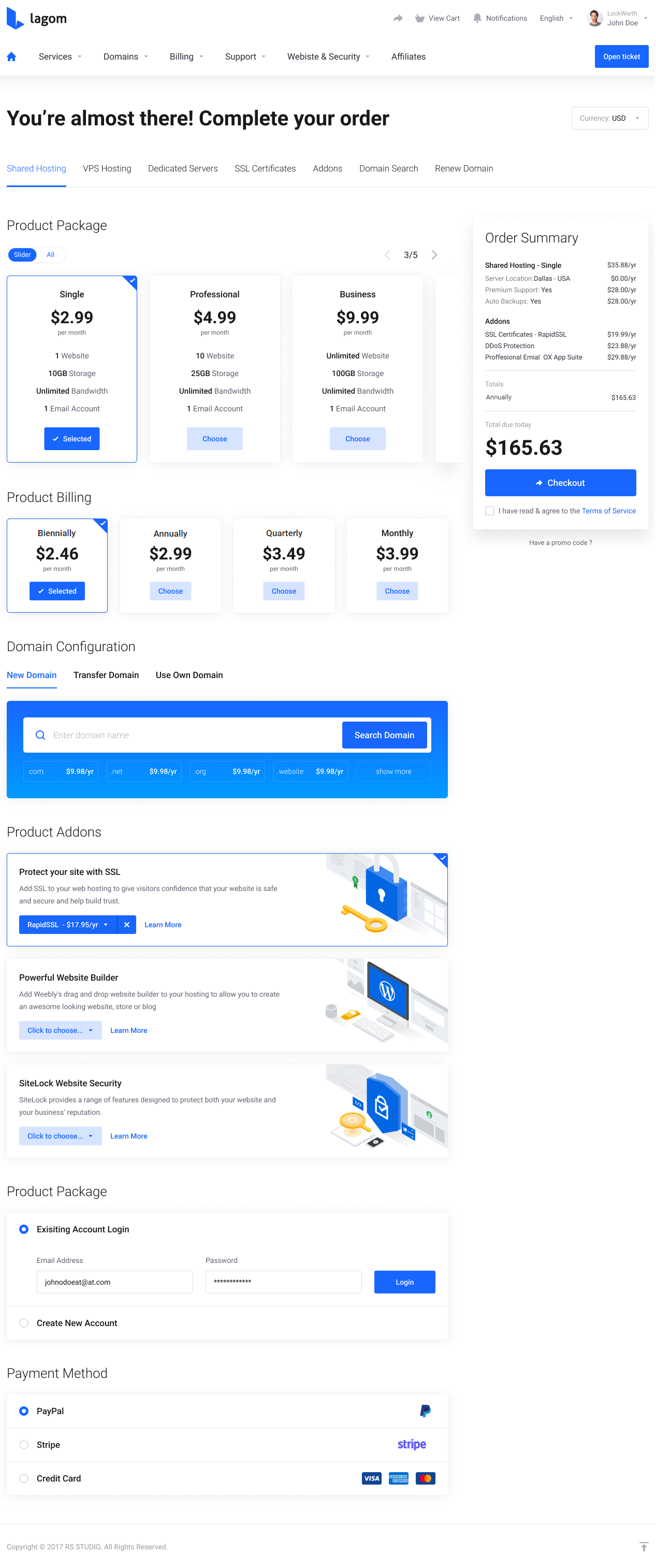The screenshot showcases a webpage that features a clean design with a white background. In the top-left corner, there's a distinctive blue logo resembling the letter "L" with a small white segment beneath it. Beside the logo, the site name "LAGOM" is clearly displayed.

On the upper-right side of the page, there's a gray text that appears distant and somewhat difficult to decipher. Adjacent to this gray text is a profile picture of a person, accompanied by their name. Left of the profile picture is a set of clickable gray buttons.

Below the person's picture, there's a blue button. Beneath the logo, a series of drop-down menus are neatly aligned. The main content area welcomes users with the message "You're almost there, complete your order" in bold black font. Below this message, users can choose from three different packages labeled Single ($2.99), Professional ($4.99), and Business ($9.99).

To the right side of the page, an order summary invoice displays a total amount of $165.63. Further down, there is a section titled "Domain Configuration" with a prominent search bar and associated drop-down menus. Under this, the "Product Add-ons" section offers several additional packages, with a few options already selected.